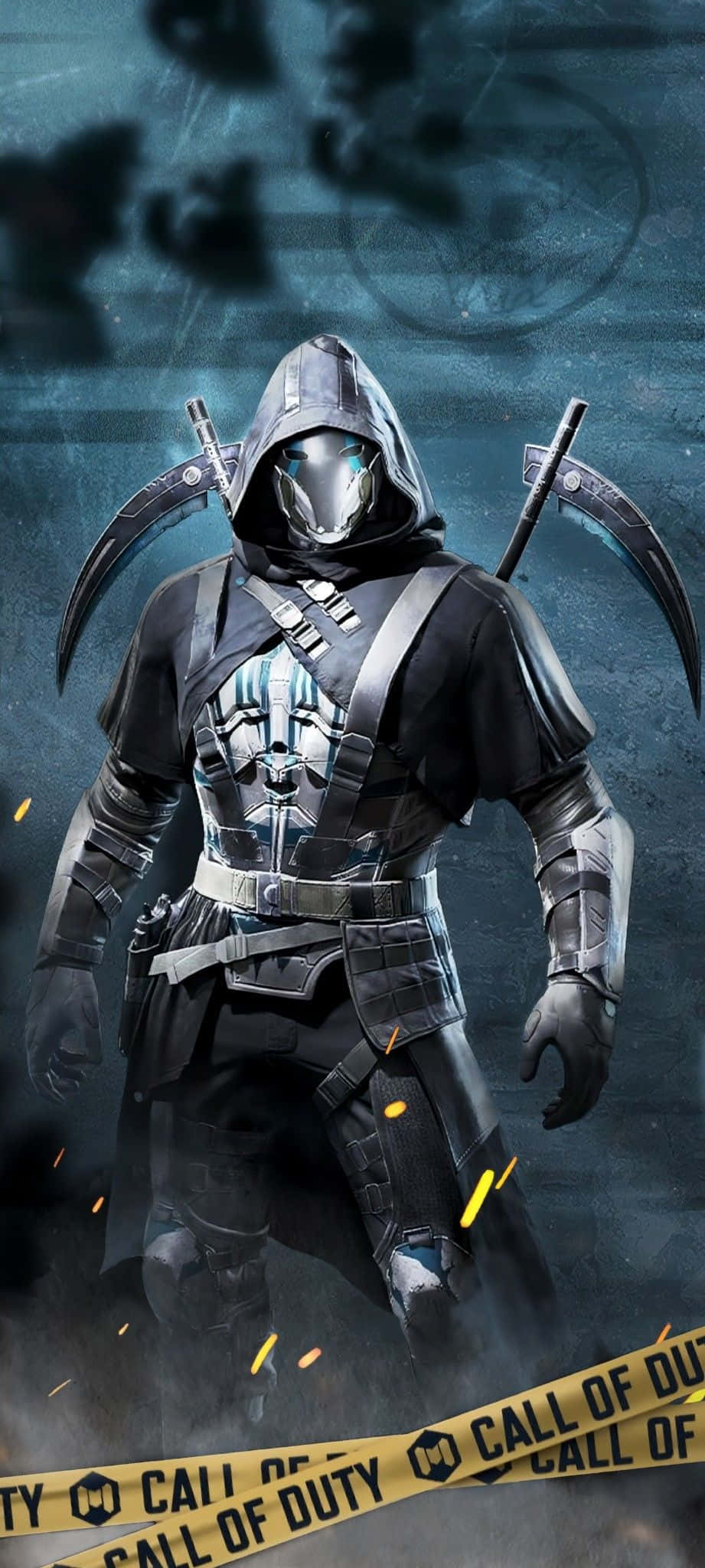This vertical rectangular image depicts a heavily armed and armored character from the video game series Call of Duty. The character stands in a dark and gritty environment that features a stormy, dark blue and gray watercolor-style background, reminiscent of a night sky with subtle sparks emerging from the bottom right. The atmosphere exudes a sense of aged, dusty grunge, contributing to the character’s menacing appearance.

In the foreground, the character is fully suited up, shrouded in a dark gray hooded cape with a metal mask that has glowing blue eyes, obscuring any visible skin. The character is equipped with numerous metal accessories, including arm guards, knee pads, belts, harnesses, and a full set of armor adorned with buckles. On their back, two crossed sickles are prominently displayed, ready for combat. The character also holds additional weaponry, including a firearm, enhancing their readiness for battle.

At the bottom of the image, two pieces of yellow caution tape are crossed and prominently display the Call of Duty logo, reminiscent of police line tape used in active investigation scenes. Above, a partially visible logo featuring a drawing of a wolf further embellishes the image, adding to the intricate and detailed artwork. The character’s poised stance coupled with the dark, tumultuous background conveys an imminent sense of action and intensity.